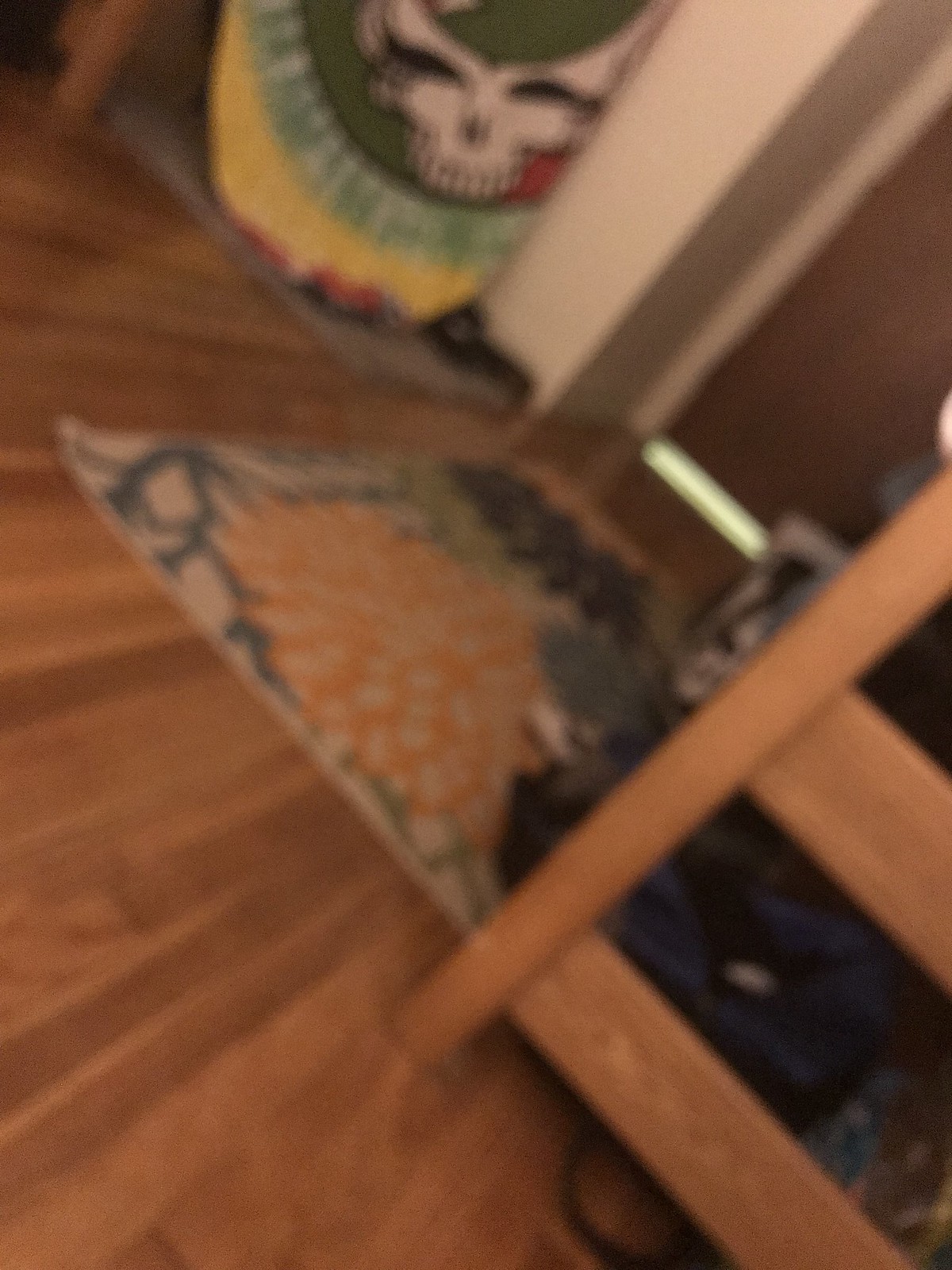In this photograph, we are presented with a view down a hallway in a modern, cozy interior. To the right, there is a partially visible wooden stand made from light-colored wood; this stand features a central vertical post with two horizontal posts extending from it. The floor beneath it contrasts slightly with a mix of light to medium wooden tones. A plush white rug featuring a vibrant floral pattern in blue, orange, and green hues occupies part of the hallway floor. On the right side of the image, a blue backpack is casually placed. The hallway leads to a dark brown door at the far end, with a sliver of light streaming from underneath it, accentuating the white walls beside it. Adding a splash of color and intrigue, a surfboard adorned in yellow, green, and red stands against the wall, decorated with a striking design: a white skull with black eye sockets.